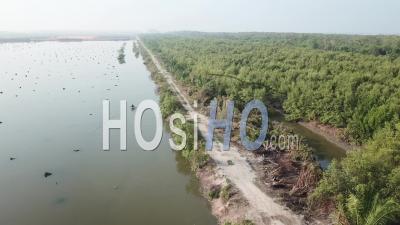This aerial photograph, branded with "HoSiHo.com" in the center, captures a sharp, straight shoreline bordered by a sandy, gravel walking path. The path runs close to a murky, brownish body of water, which is likely man-made due to its precise right-angled edges. The water appears to contain some floating debris or reflections, though its pixelated quality makes it hard to discern. On the other side of the path lies a dense area of vibrant green evergreen trees, shrubs, and brush, forming a lush, waterside greenery. In the far distance, the shoreline extends straight out to the left while the greenery continues to the right. The sky, visible in parts of the image, appears light blue but overexposed. There are also occasional boulders dotting the water's surface. Overall, the photo presents a peaceful outdoor landscape devoid of human presence.